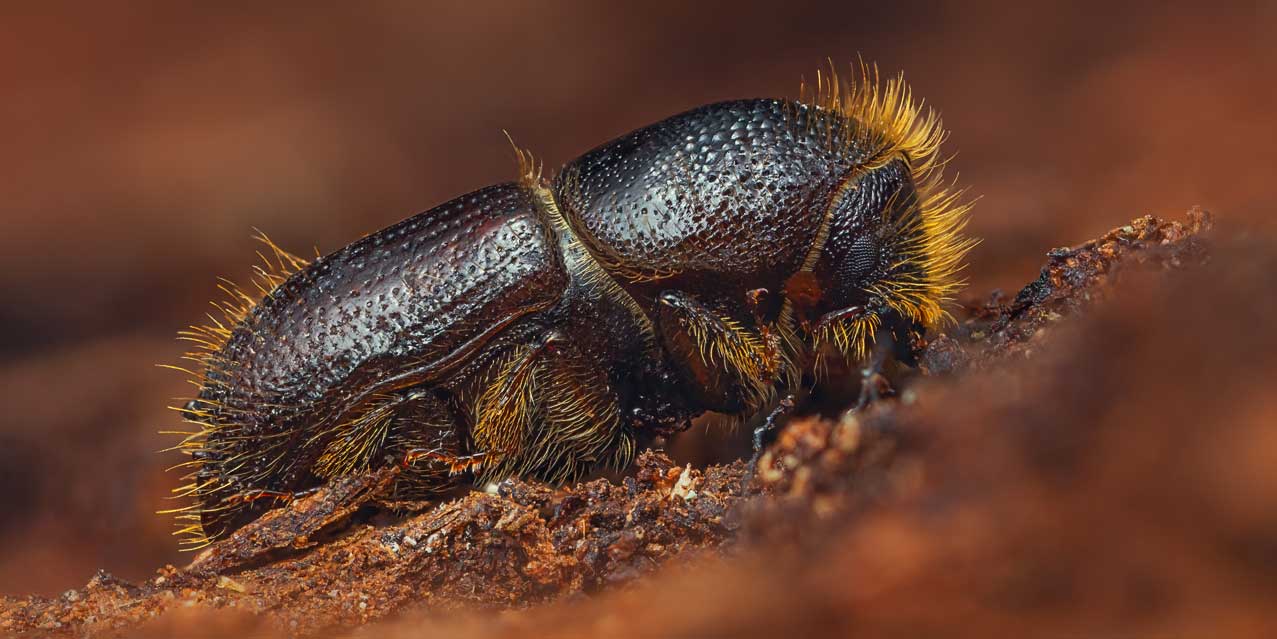This is a high-definition, close-up photograph of an insect situated on a light brown, blurry background, which appears to be either soil or a branch. The insect occupies almost the entire frame and has a distinctive dark brown to black, shiny, and hard exterior. Its body structure is somewhat ambiguous, resembling a snail without its shell or a peanut due to a unique middle part that protrudes like an arm. The insect is covered in fine yellow-orange hairs, particularly noticeable along its top and back. These straight, thin hairs contrast with the insect's glossy surface, adding a textured detail to its appearance. The insect is curled in on itself, making it challenging to identify its head or backside.